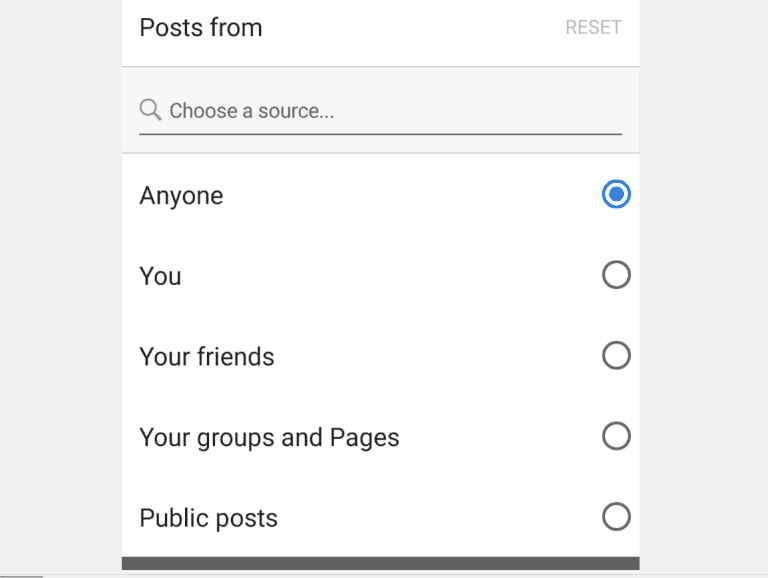The image depicts a neatly designed drop-down menu from a social media platform, intended for users to filter posts by source. At the top center, a label reads "Post From," immediately followed by a search bar spanning the width of the dropdown, with placeholder text stating "Choose a Source." 

Beneath the search bar, there are six selection options arranged vertically: "Anyone," "You," "Your Friends," "Your Groups and Pages," "Public Posts," and "Custom." Each option has an adjacent button on the right side. The selected option, "Anyone," is indicated by a filled blue dot, while the remaining options have empty circles, signifying they are not selected. 

In the faintly visible top right corner is a "Reset" option, presumably for clearing all selections. Structurally, the drop-down menu has a light gray outer background, with a white interior that ensures the dark gray text is easily readable. The overall color scheme is minimalist, featuring primarily white and gray tones, with blue used effectively to highlight the active selection.